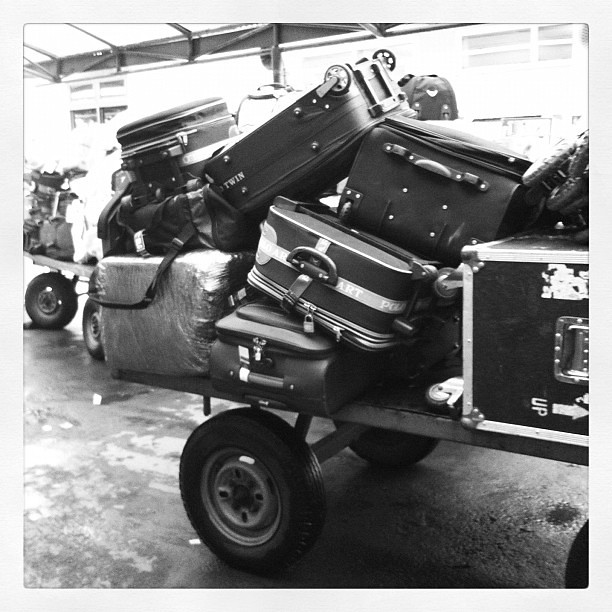The black and white image depicts a chaotic scene of luggage piled atop a trolley with a flat platform and two visible large tires. The main cart is overloaded with around seven suitcases of various shapes and designs, some featuring black and white stripes. Among the suitcases, there is a black box with silver borders and an 'up' label pointing to the right, as well as a mysterious plastic-wrapped item that appears softer and squishier than the other luggage. The ground beneath the trolleys appears wet, suggesting a cement or asphalt surface. In the background, another similar trolley can be seen, also laden with luggage, beneath a metal covering or awning. Behind this, a building with windows is partially visible, adding to the industrial ambiance of the scene. The photo, encased in a white border, captures a moment that could be from an airport or a similar transit hub, although no specific location is indicated.